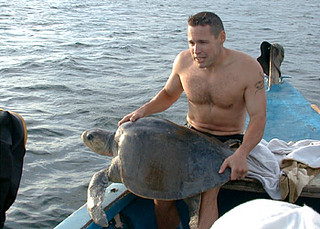In the photograph, a shirtless man wearing black swim trunks sits on a bench aboard a blue, slightly dirty boat, holding a large gray sea turtle in his lap. The turtle, with its head and fins clearly visible and facing left, is illuminated by a bright light source highlighting its flippers and shell. Multiple white and brown towels are scattered around where the man is seated. Behind him, you can see the choppy gray and blue waves of a large body of water, indicating some level of wave action. Towards the front of the boat, a large rod intertwined with multiple ropes is visible. In the bottom left corner of the image, a person with a camera is capturing the scene, contributing to the dynamic atmosphere of this outdoor shot.